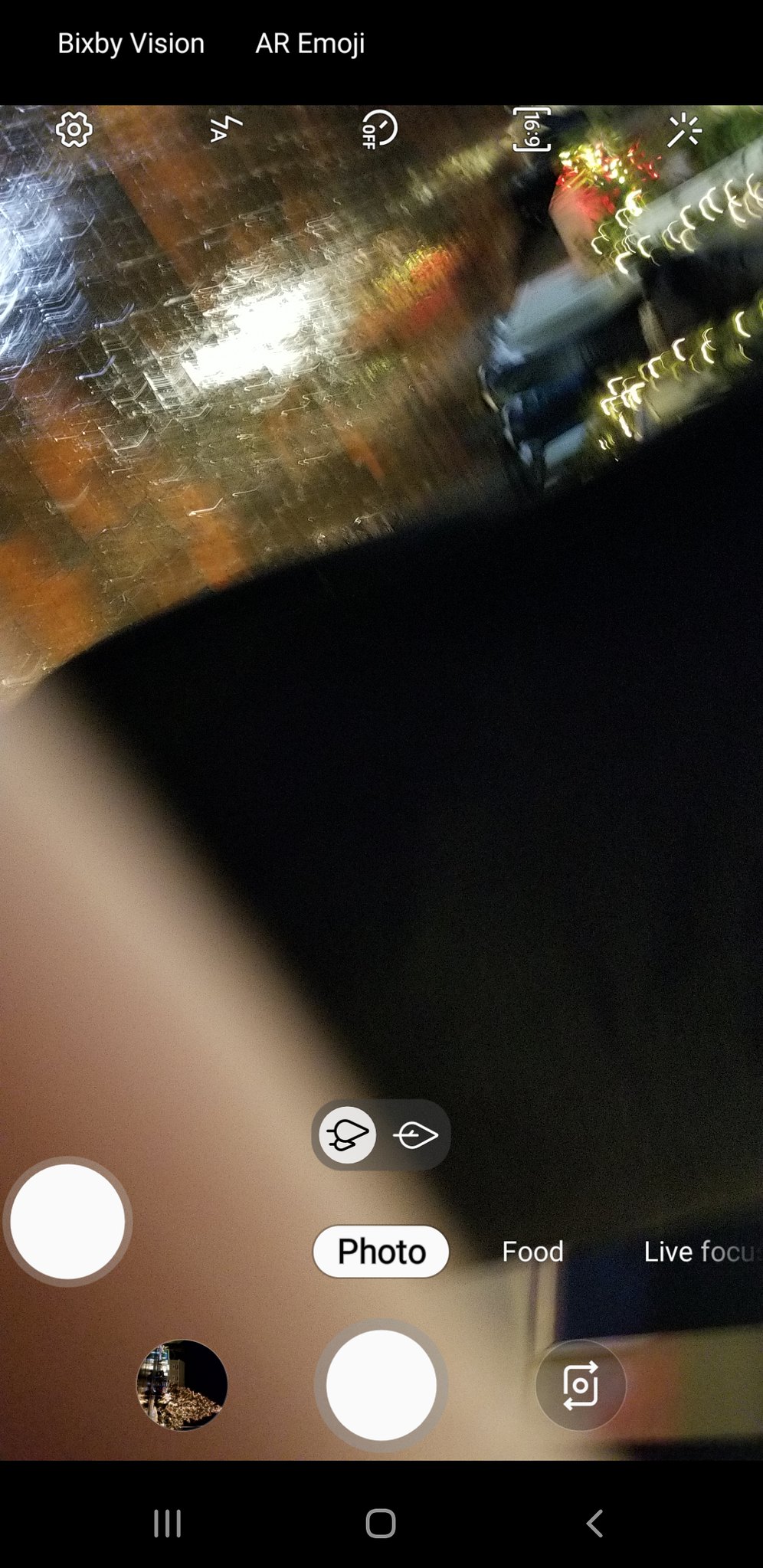This is a vertical screenshot of a smartphone's camera interface. At the top and bottom of the image are black bars typical of a phone's display layout, creating a letterbox effect. The top bar features options in white text, including "Bixby Vision" and "AR Emoji." The bottom bar contains various camera mode icons and buttons in white and grey. 

The central portion of the screenshot displays an out-of-focus photograph being taken, dominated by a reflective gold object towards the top of the frame. A blurry arm is visible in the bottom left corner. The area around the arm appears white and indistinct.

On the lower part of the screen, there's a circular white button for capturing photos, flanked by text options such as "Photo" directly above it, and "Food" to the right. Further to the right, "Live" can be partially seen. Additionally, there are several circular icons along the top of this lower section: one white circle slightly to the left, another circular icon below it, and to the right, a camera icon within a circle.

Overall, this screenshot captures the moment a user is in the process of taking a photo using various available camera options and features on their smartphone.